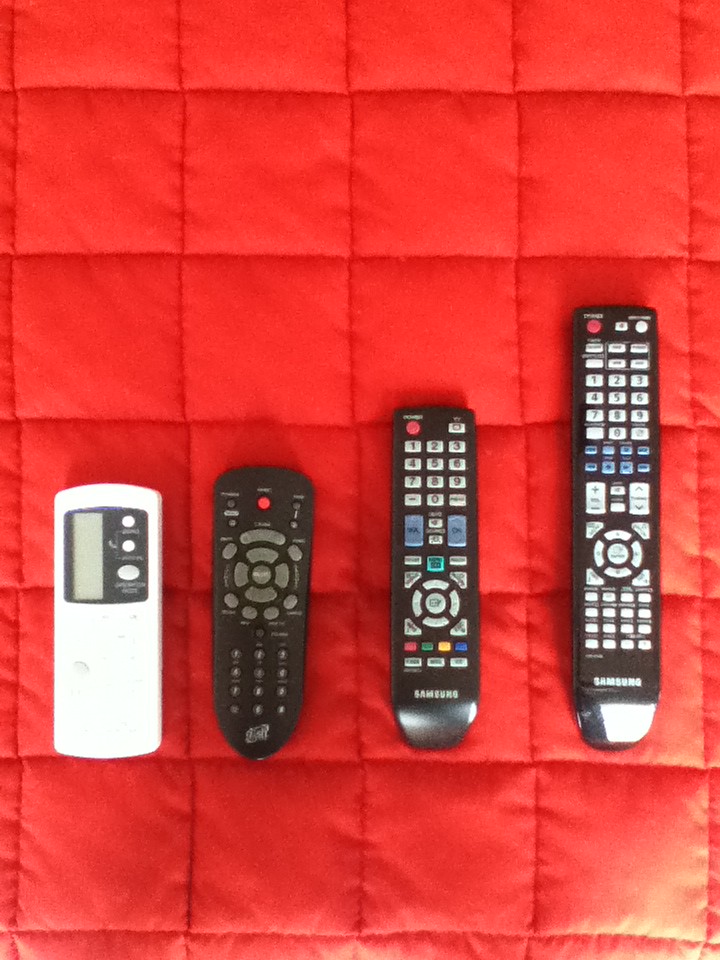The image captures a photographic perspective from above, showcasing a vibrant red quilt or blanket designed with a grid-like square pattern. Arranged neatly on this textured quilt are four remote controls, positioned side-by-side in ascending order of size. Beginning from the left, the first device is a white remote with a vertical screen and three buttons. Next to it is a small, oval-shaped remote which is predominantly black, featuring gray buttons with a lone red button at the top. The third remote in line is slightly larger and more colorful, sporting buttons in red, blue, green, yellow, gray, and teal hues. The final remote is the largest, rectangular in shape and primarily black, adorned with various buttons in white and blue, with a distinctive red button at the top. The bottom section of the quilt displays a soft yellow reflection, adding a subtle highlight to the scene.